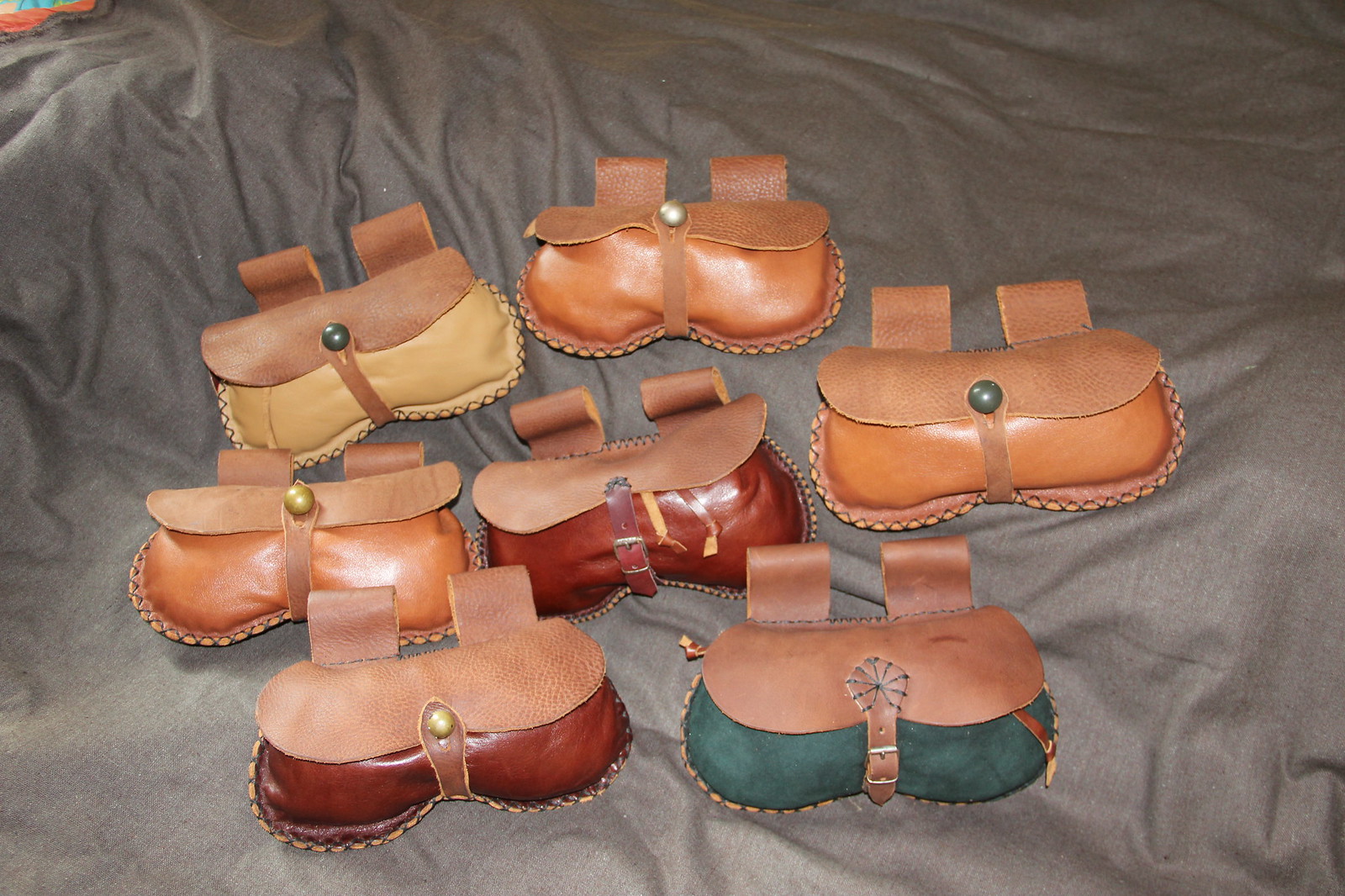The image showcases seven handmade leather satchels arranged on a gray felt sheet. Each satchel features distinct colors and styles, sharing a uniform design with top loops likely for attaching to belts. The satchels, which resemble large leather glasses cases, exhibit a shiny finish that reflects the light, highlighting their texture. The top sections, mostly tan, close with either button snaps or buckles and include straps for securing the satchels. The bottom sections vary in color, including green, maroon, and multiple shades of orange and tan. The arrangement consists of two satchels at the back (one yellow and one orange), three in the middle row (an orange flanked by a red and another orange), and two in the front (a red and a green). The distinctive materials, including smooth leather and suede textures, add to the unique appeal of each piece, making them practical belt bags or fashionable accessories.